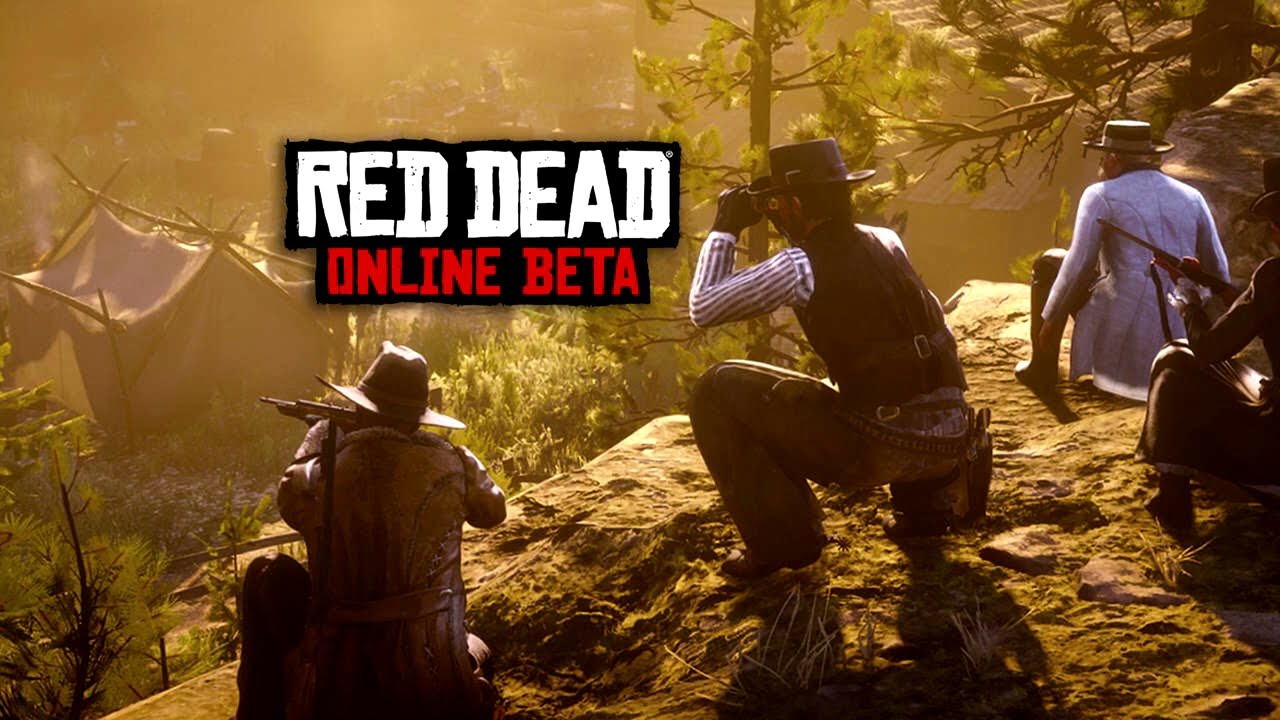The image is a detailed screenshot from a video game, specifically an advertisement for "Red Dead Online Beta." It depicts a western-themed setting with four characters standing and crouching on the edge of a ridge overlooking a valley below. The characters are dressed in traditional cowboy attire, featuring leather vests, hats, and boots. The leftmost character, wearing a top hat and a greenish-brown cloak, holds a rifle aimed down to the left. The next character, closer to the camera, sports a striped shirt, leather vest, and black gloves, and uses binoculars to survey the area. Only part of the third character is visible, dressed in all black and carrying an assault rifle, their left knee and arm, and a black hat showing. The rightmost character, wearing a white long cloak and brown boots, also aims a gun downwards. The valley below is dotted with light-colored canvas and wooden tents amid green grass and sparse trees. The sky exhibits a brownish-red hue, giving the scene a distinct atmospheric tension. Text across the image reads "RED DEAD" in white, followed by "ONLINE BETA" in red font at the top.